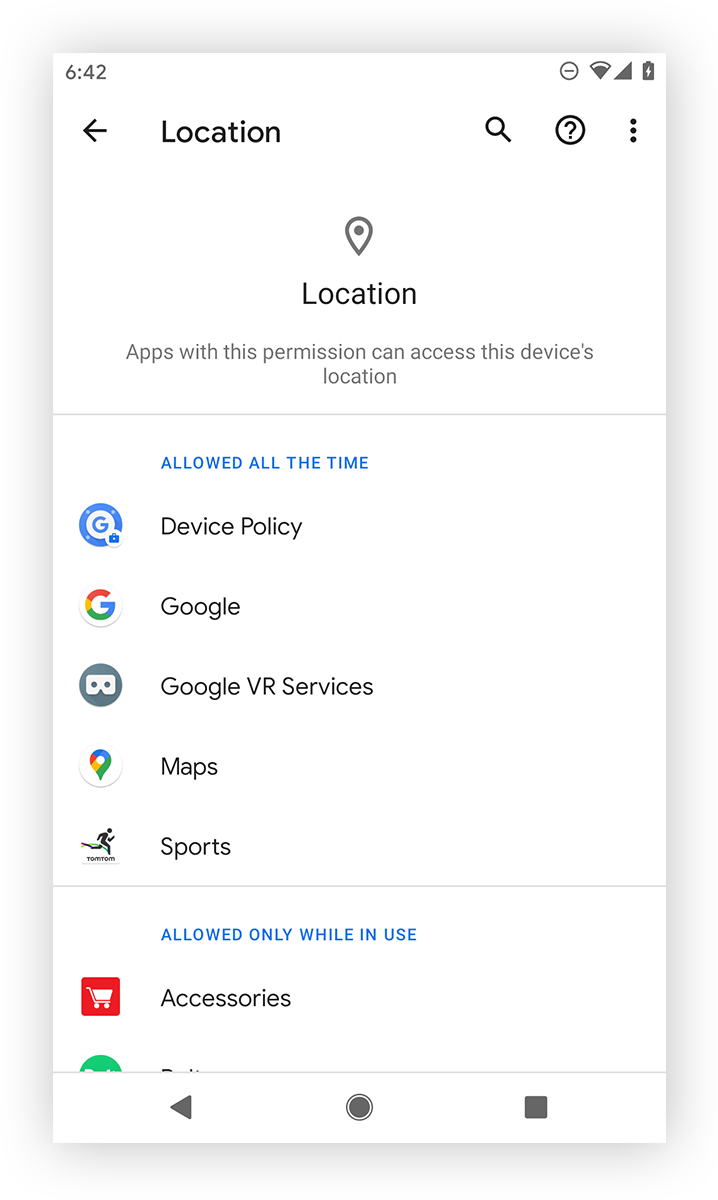A screenshot of an Android smartphone's settings menu emphasizes location permissions. The screen, with a white background and black text, shows the top status bar displaying the time as 6:42 (AM/PM not specified), cell signal strength, Wi-Fi connection, and remaining battery power. This section of the settings menu is specifically for location permissions, detailing which applications can access the device's location. At the top, a message states, "Apps with this permission can access the device's location." Below, a list of applications with full location access is visible: Device Policy, Google, Google VR Services, Maps, and Sports. Additionally, a subcategory under this list shows apps that can access the location only while in use, with "Accessories" partially visible among other applications. The screen also features an option to search settings, ask questions, and navigate through different pages.